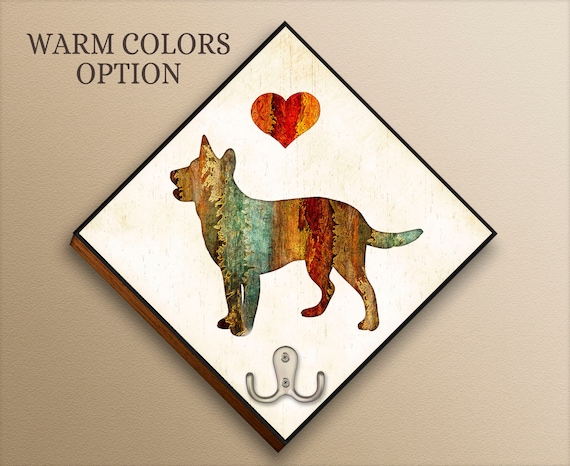This image showcases a rustic home decor sign, square in shape but rotated 45 degrees to appear as a diamond. The background is a gradient from darker brown in the lower left to lighter shades in the upper right. At the center of the sign, against a rustic white background framed by a brown outline, there are vivid multicolored images: a red and orange heart at the top and a striped silhouette of a dog or wolf in shades of brown, green, red, gold, blue, and aqua facing left. Below these images, a silver coat hook with a dual prong design and rounded attachment is secured with two screws. In bold, uppercase brown letters, the top of the sign reads "WARM COLORS" followed by "OPTION." This piece appears to be an advertisement or sample showcasing different warm color options.